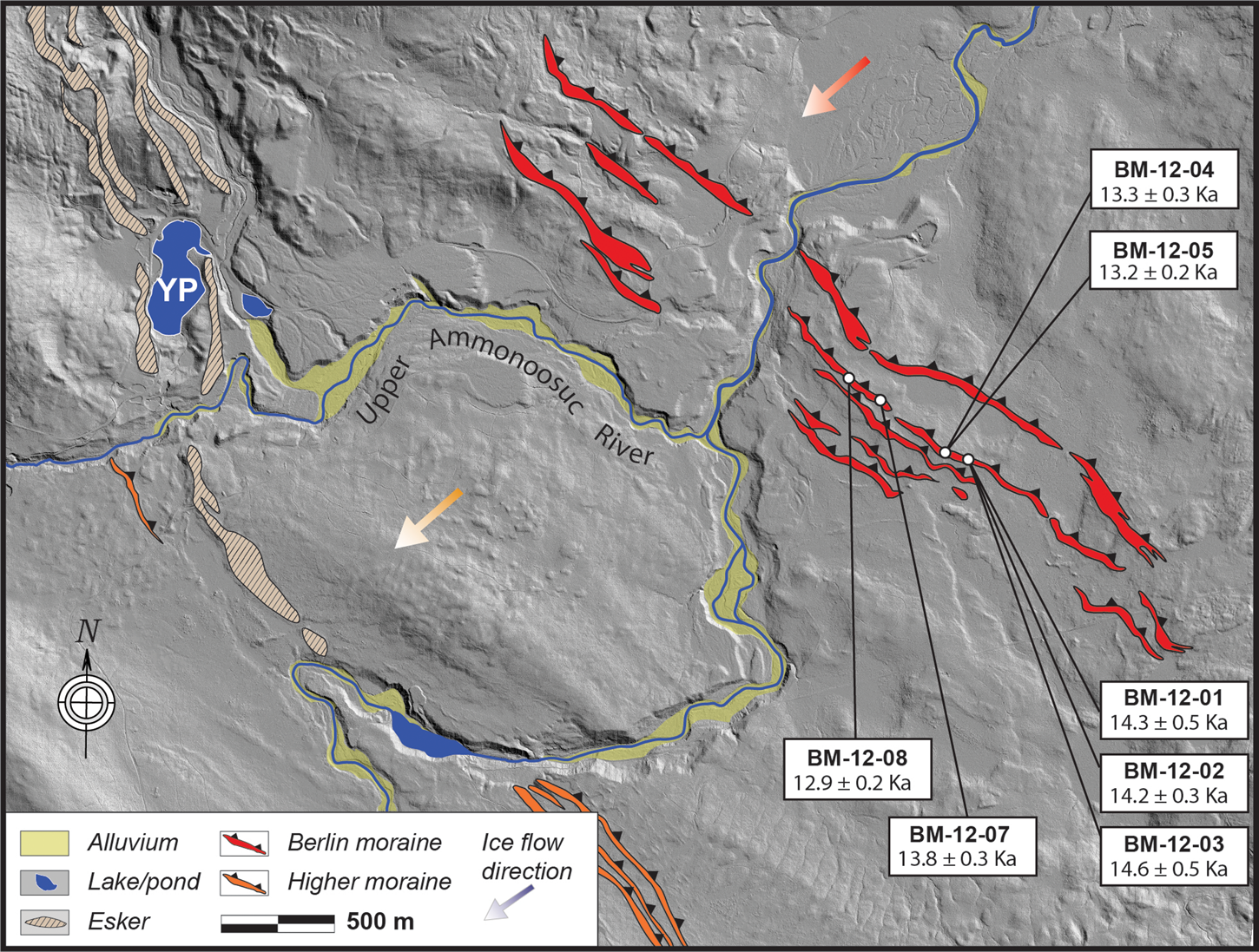This image is an overhead view of a topographical map, primarily gray in color, depicting a detailed representation of the upper Aminozoic River area. The map features a color-coded guide in the bottom left corner, explaining various natural elements: green for alluvium, blue for lakes and ponds, brownish-striped for esker, red for Berlin moraine, and orange for higher moraine. A prominent green strip of alluvium starts from the left, curves downward, and moves back to the left, intersecting a blue-marked pond at the bottom and another pond labeled with "YP" at the top left. The esker originates from the top left corner, descending past the pond. The Berlin moraine, depicted in red, stretches from the top, moving left to right and curving downward across the right side. The higher moraine, marked in orange, is visible in the bottom center. An arrow indicating the ice flow direction points southwest, while black lettering in the map's center reads "upper Aminozoic River," accompanied by an orange arrow also pointing southwest. Several white boxes on the right contain the annotations "BM-12-08," "BM-12-04, 13.3 ± 0.3 Ka," and "BM-12-05, 13.2 ± 0.2 Ka," with arrows pointing towards the red Berlin moraine. A north directional compass is present, confirming the map's orientation.